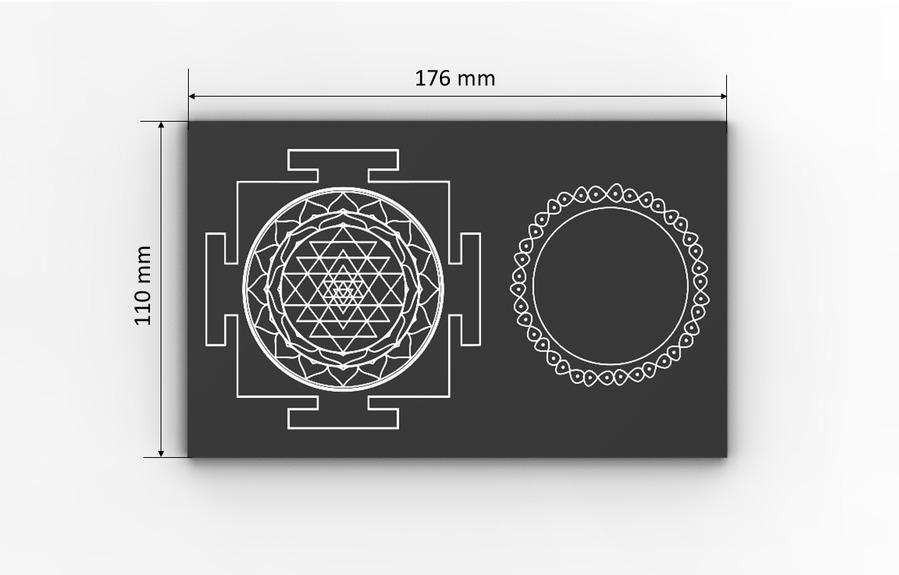This detailed black-and-white image features two distinct scroll designs, set against a gray background. On the left side, there is a decorative circular motif surrounded by triangles and boxes, creating an intricate, almost floral pattern. On the right side, a similar circular design is embellished with petal-like shapes encircling it. The image also includes precise measurements: "176 millimeters" is labeled at the top with arrows extending in both directions, and "110 millimeters" is marked on the left side, also with bidirectional arrows. This visual composition blends geometric and floral elements, rendered in monochrome for a striking effect.